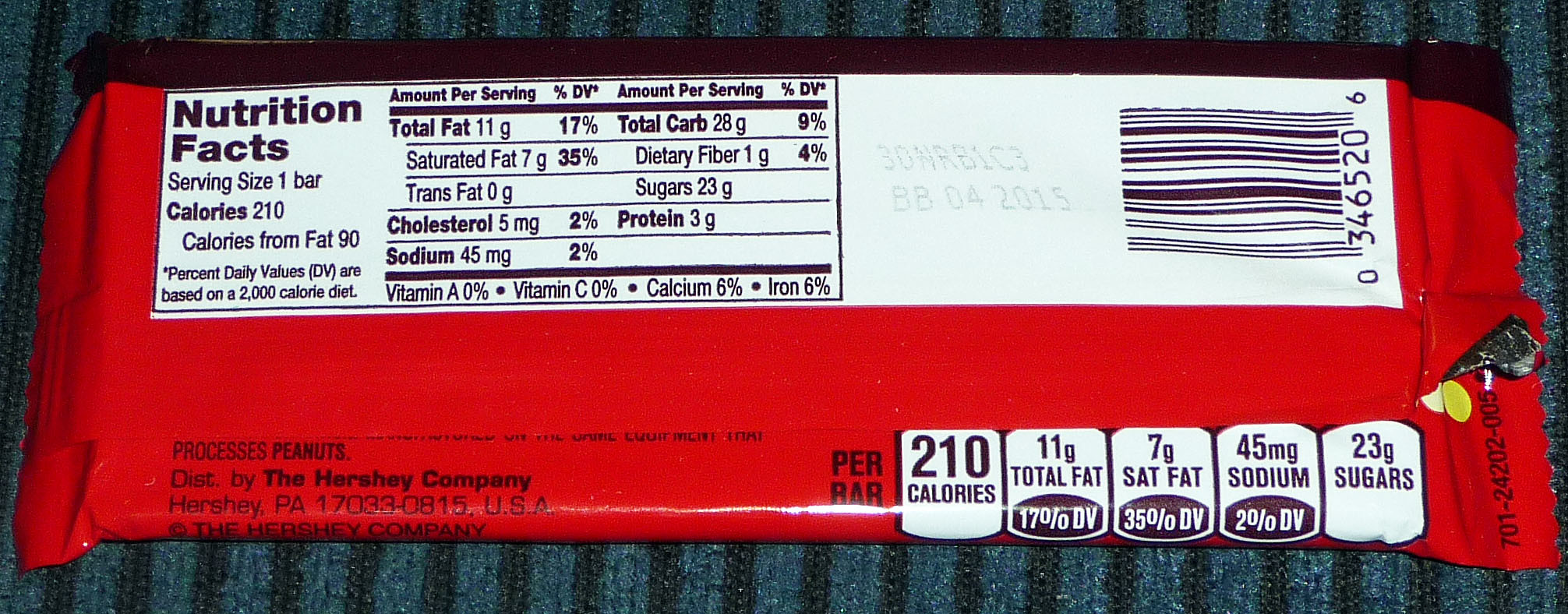In this highly zoomed-in image, the focus is on the backside of a red candy bar wrapper. The left side of the image features the outer edges of the packaging, showcasing the predominantly red color scheme. On the right, a white area surrounds the Nutrition Facts label, providing contrast against the red background. The top section of the candy bar is cast in shadow, appearing dark brown.

The Nutrition Facts label details that one serving size is 1 bar, containing 210 calories, with 90 calories from fat. This information is positioned on the left side of the label, while the various nutrients and their respective percentages are listed to the right. Below this, the levels of Vitamin A, Vitamin C, Calcium, and Iron are stated, with Vitamins A and C both at 0%, and Calcium and Iron at 6%. To the right of these details is a white rectangular section featuring a barcode.

Beneath the barcode are five additional labels providing further nutritional information. The entire candy bar wrapper rests on a surface characterized by a pattern of blue and black stripes, which may be part of a cloth or fabric.